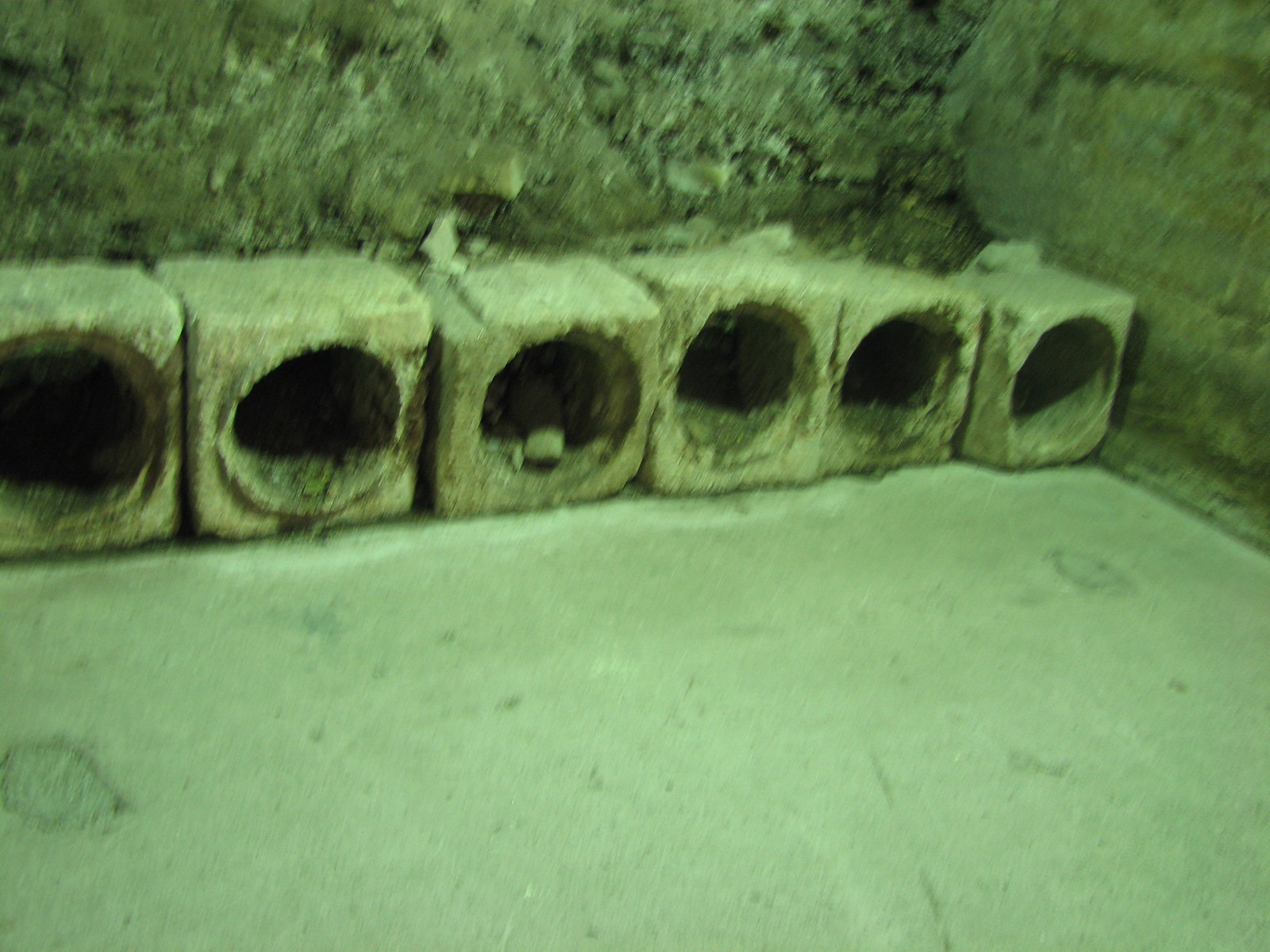The image depicts an old, cracked, and weathered concrete structure, featuring rough, hole-riddled walls that intersect at a corner in the upper middle right side. The concrete floor, while slightly smoother than the walls, still displays signs of age and wear. Positioned against the back left wall are six square concrete blocks, each with large circular holes bored through them, possibly serving a drainage function. This scene resembles an empty canal or overflow area, where water from these perforated blocks typically drains and fills the space. The entire setting exudes a sense of enduring antiquity through its chipped and eroded surfaces.